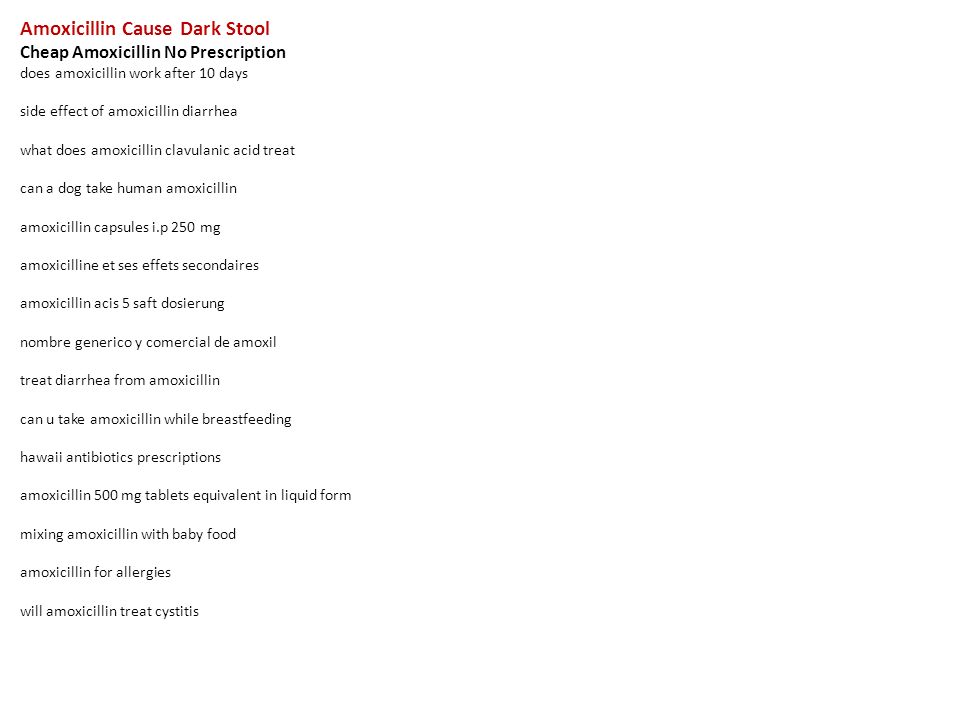The image features a text on a white background with a prominent red heading at the top reading, "Amoxicillin Called Dark Stool." Below the heading, in bold black letters, it states, "Cheap Amoxicillin, No Prescription." Following this, in non-bold black letters, there is a series of questions and statements related to the use and effects of amoxicillin:

- "Does amoxicillin work after 10 days?"
- "Side effect of amoxicillin: Diarrhea."
- "What does amoxicillin with clavulanic acid treat?"
- "Can a dog take human amoxicillin?"
- "Amoxicillin capsules I.P 250 MG."
- "Amoxicillin extended-release effects secondary."
- "Amoxicillin assist 5-stop dozy room."
- "Nombre generico de amoxicillin."
- "A commercial de amoxo."
- "Treat diarrhea from amoxicillin."
- "Can you take amoxicillin while breastfeeding?"
- "Hawaii antibiotics prescription."
- "Amoxicillin 500 mg tablets equivalent in liquid form."
- "Mixing amoxicillin with baby food."
- "Amoxicillin for allergies."
- "Will amoxicillin treat cystitis?"

Overall, the image appears to be a visually cluttered advertisement or informational graphic about various aspects of amoxicillin, addressing questions and issues related to its use in both humans and animals.